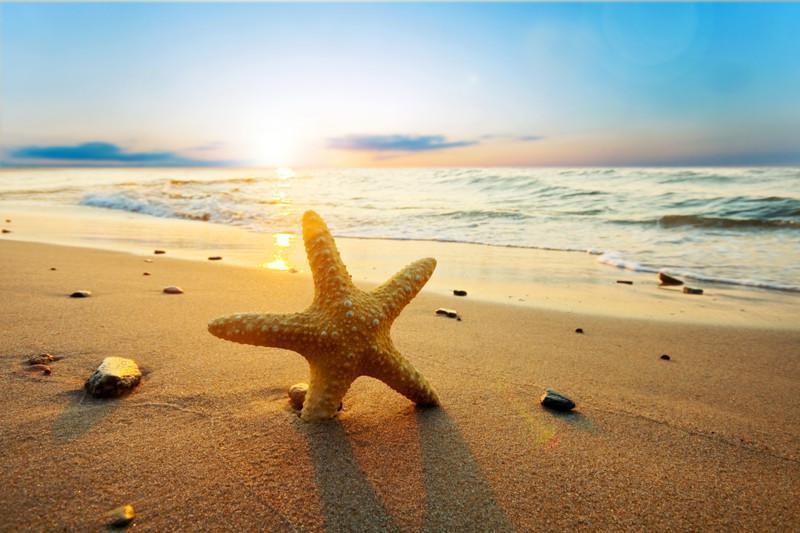The photograph depicts a serene and peaceful beach scene at either sunset or sunrise, featuring a starfish prominently standing upright in the foreground. The starfish is golden in color with cream-colored bumps, and one of its legs is deeply submerged in the sand, giving it a vertical stance while the other legs extend outward. Surrounding the starfish are scattered pebbles and shells, adding texture to the sandy shore. The ocean, depicted as calm with barely any cresting waves, glows with the reflection of the sunlight. The receding water line glistens, indicating a recent wave retreat. The sun, positioned at the horizon, shines brightly, casting a white glow that reflects off the wet sand, creating a doubling effect. The sky above features a beautiful gradient of pinks and blues with a few scattered clouds, contributing to the overall tranquil ambiance of the scene.